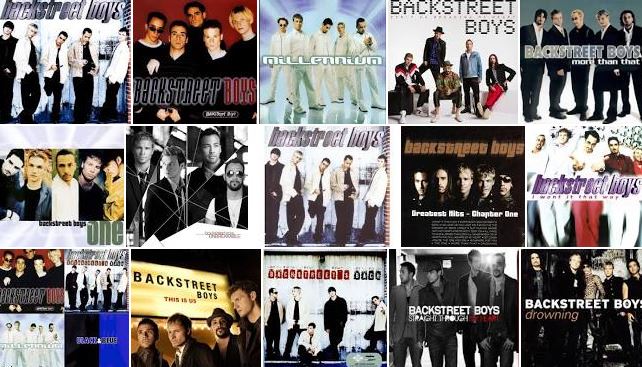The image displays a grid of 15 compact disc covers showcasing the discography of the Backstreet Boys, arranged in three rows of five. Each cover features the band's name prominently, often in different colors, depicting the five members in various poses and settings. Some covers highlight the members against solid maroon walls or external brick walls, while others show them in motion, walking down hallways or alleys. The members' outfits vary, including black shirts and pants paired with white or tan jackets. Notable album titles include "Millennium" and "One." The covers collectively reflect the band's evolving aesthetic over time, with close-up headshots and group shots in various dynamic scenarios, including one where they stand in front of a theater sign displaying their name.